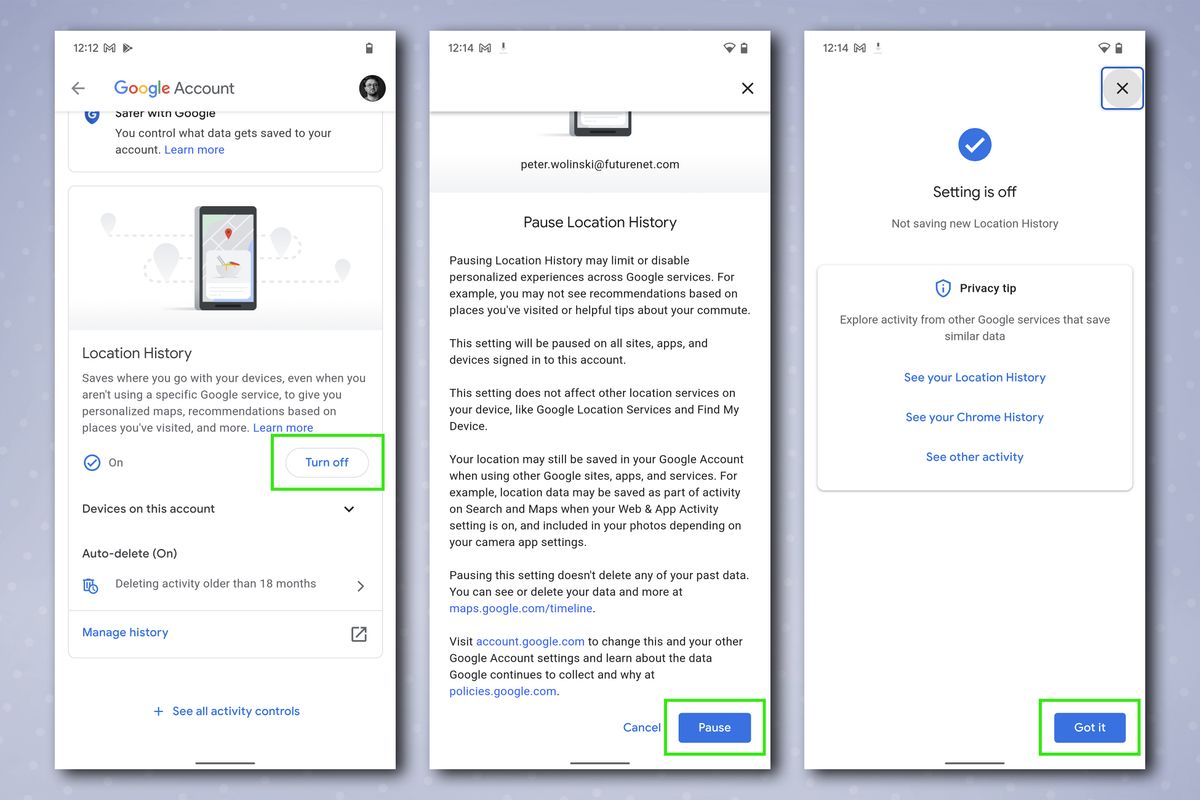Here's the cleaned-up and detailed caption for the image:

---

The composite image features three horizontally aligned screenshots on a light gray background, each displaying different stages of a Google Account settings page on a mobile device. Each screenshot has a white background and timestamped headers, indicating times around 12:12 to 12:14, along with various symbols in the status bar, including Gmail, downloading indicators, Wi-Fi strength, and battery icons.

**First Screenshot (12:12 PM):**
- **Header:** Contains the Gmail icon followed by a partially filled arrow, indicating an ongoing download, and symbols for Wi-Fi and battery status.
- **Title:** "Google Account. Safer with Google. You control what data gets saved to your account." There's a "Learn more" clickable link in blue.
- **Avatar:** A black and white avatar of a presumed male figure wearing glasses is located in the upper right corner.
- **Content:** Features an icon of a cell phone overlaid with a red location symbol and text explaining the function of Location History, which saves places visited even when not using Google services, to provide personalized recommendations.
- **Settings:** Currently, Location History is turned ON (indicated by a blue toggle on the left), with options such as "Devices on this account" with a dropdown arrow, "Auto-delete on" for deleting activities older than 18 months, and "Manage history" and "See all activity controls," both in blue.

**Second Screenshot (12:14 PM):**
- **Header:** Similar to the first, with the Gmail icon, half-colored download arrow, Wi-Fi, and battery symbols.
- **Email:** Displayed is "peter.wolinski@futurenet.com."
- **Title:** "Pause location history."
- **Explanation:** Details the impact of pausing Location History, including the potential limitations on personalized experiences across Google services and how location data might still be saved in various circumstances.
- **Links:** Includes "maps.google.com/timeline" and "account.google.com" in blue for viewing and managing data, as well as "policies.google.com" in light blue for understanding data collection policies.
- **Actions:** Options to "Cancel" in blue and a prominently outlined "Pause" button, indicating a suggested action to pause Location History.

**Third Screenshot (12:14 PM):**
- **Header:** Mirrors the symbols of the second screenshot, indicating status bar consistency.
- **Canceled Action:** Features a grayish circle with a black 'X' and a blue outline, suggesting an undo or cancellation prompt.
- **Central Info:** Displays a blue circle with a white tick and the message "Setting is off, not saving new location history."
- **Privacy Tip:** Contains a shield symbol with a blue eye, providing information on exploring similar data saved by other Google services. Hyperlinks to "See your location history," "See your Chrome history," and "See other activity" are provided.
- **Acknowledgment Button:** A blue rectangle outlined in green with "Got it" in white, placed at the bottom right, indicating a confirmation action.

---

This detailed caption encompasses the visual and textual details presented in the screenshots comprehensively.